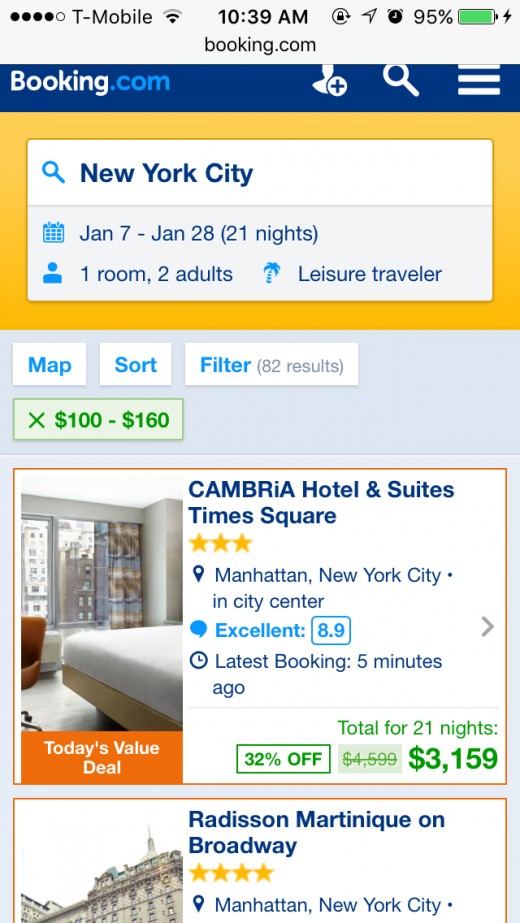Screenshot of a mobile device displaying a Booking.com webpage details:
 
The screenshot, taken at 10:39 a.m. with a phone connected to the T-Mobile network at 95% battery, shows the Booking.com app interface. The top banner of the app, in a purple-blue hue, contains a generic user icon with a plus sign, a search bar, and a menu icon represented by three horizontal lines. Below this, the search details specify a trip to New York City from January 7th to January 28th for a total of 21 nights, searching for one room accommodating two adults, identified as leisure travelers.
 
The interface further includes interactive white boxes for map view, sorting options, and filters. The selected price range filter indicates a nightly rate between $100 and $160. Two hotel options are visible: Cambria Hotel and Suites in Times Square, which holds an excellent rating and a total cost of $3,159, and Radisson Martinique on Broadway, displaying a four-star rating, although its price is not fully visible due to the screen cutoff.